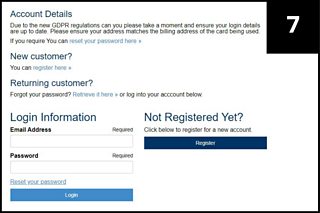The screenshot displays a web interface for an account login and registration system. The layout features a predominantly white rectangular section outlined in black. In the top right corner of this section, there is a solid black square with a white number '7' inside it.

On the left side, the heading "Account Details" is prominently displayed in blue. Below this heading, a paragraph of text is written in black, providing further details. Another blue header reads "New Customer?" followed by an invitation to register, with a link provided.

For returning customers, there is a prompt titled "Returning Customer?" which asks for a password and includes a link to retrieve it if forgotten. The section includes input fields for email address and password, followed by a 'Login' button.

Towards the bottom, a message reads "Not registered yet?" with an accompanying link directing users to register for more information.